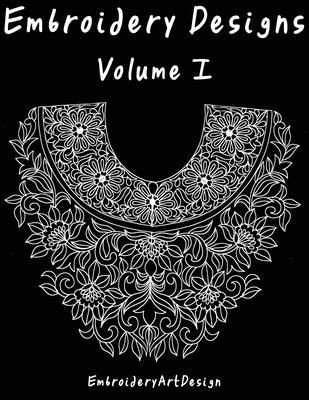The image is an advertisement for an embroidery design book titled "Embroidery Designs Volume 1" by Embroidery Art Design. It features a black background with all text in white, designed to create a stark contrast that highlights the detailed artwork. At the top of the image, "Embroidery Designs" is prominently displayed, followed by "Volume I," with the Roman numeral for one. At the bottom, the text reads "Embroidery Art Design."

The central visual element of the cover is an intricate, monochromatic embroidery pattern. The design appears to be pencil-drawn and features an array of flowers, leaves, and geometric shapes, meticulously arranged to mirror each other, suggesting a harmonious, symmetrical design. The artwork is reminiscent of a detailed breastplate or the top part of a shirt or vest, complete with a neckline, which doesn’t extend beyond the image as it is a flat illustration. The floral motifs include daisies and possibly other swirling flowers and leaves, adding to the ornate and sophisticated appearance. The overall aesthetic of the cover is simple yet elegant, focusing exclusively on the black-and-white embroidery design without any additional images or colors.